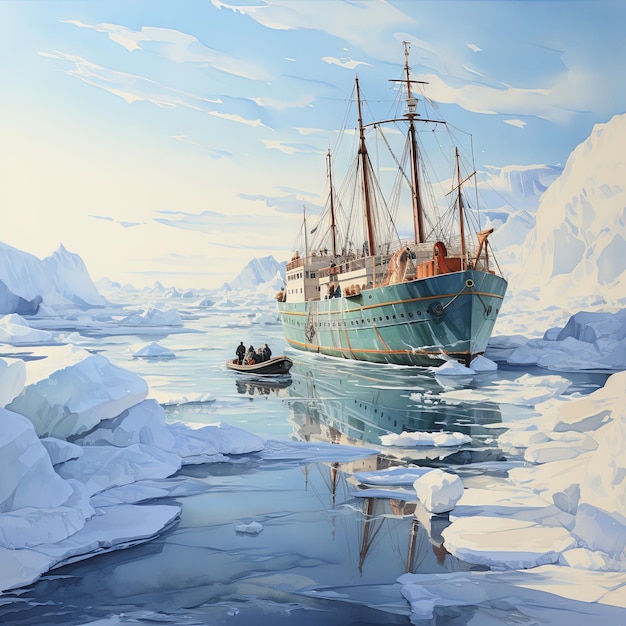The image depicts a detailed and surreal digital painting of an 18th-century style sail ship navigating through an icy, glacier-filled Arctic or Antarctic landscape. The art portrays a large, old-fashioned sail ship with prominent masts but no visible sails, painted in shades of blue with orange accents around its top and bottom, and a black hull at the very bottom. The vessel appears to be cutting through broken ice, suggesting an icebreaker may have paved its way. To the left of the ship is a small rowboat, possibly motorized, carrying about half a dozen people, with additional figures potentially visible on the larger ship, though the image is slightly blurry. The surrounding environment features towering white glaciers on both sides, casting shadows on the clear, ice-covered water beneath. The sky above transitions from a bright blue near the ship to a whiter hue in the distance, capped with white clouds, enhancing the cold, crisp atmosphere of the scene. The painting itself is square, approximately four to five inches in both height and width, amplifying the intimate yet expansive feel of this icy maritime adventure.